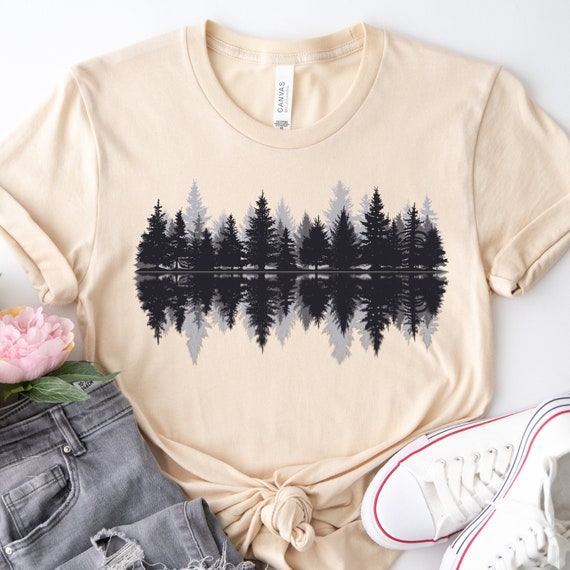In the center of this photo is an off-white t-shirt with rolled-up sleeves, artfully tied in a knot at the bottom. This shirt features a striking graphic on the front, depicting a horizon of dark, symmetrical pine trees reflected below, as if mirrored in water. The background of the image is bright and white, enhancing the clean lines and details of the apparel.

To the left of the t-shirt, a light pair of jeans is casually folded, showcasing a stylish hole at the knee. On the right, a pair of pristine white tennis shoes with red detailing just above the sole sits neatly tied. The impeccable condition of the shoes highlights their fresh, out-of-the-box look.

This composition, with its crisp and well-lit background, presents a trendy and cohesive outfit, ideal for an advertisement or clothing company promotion.